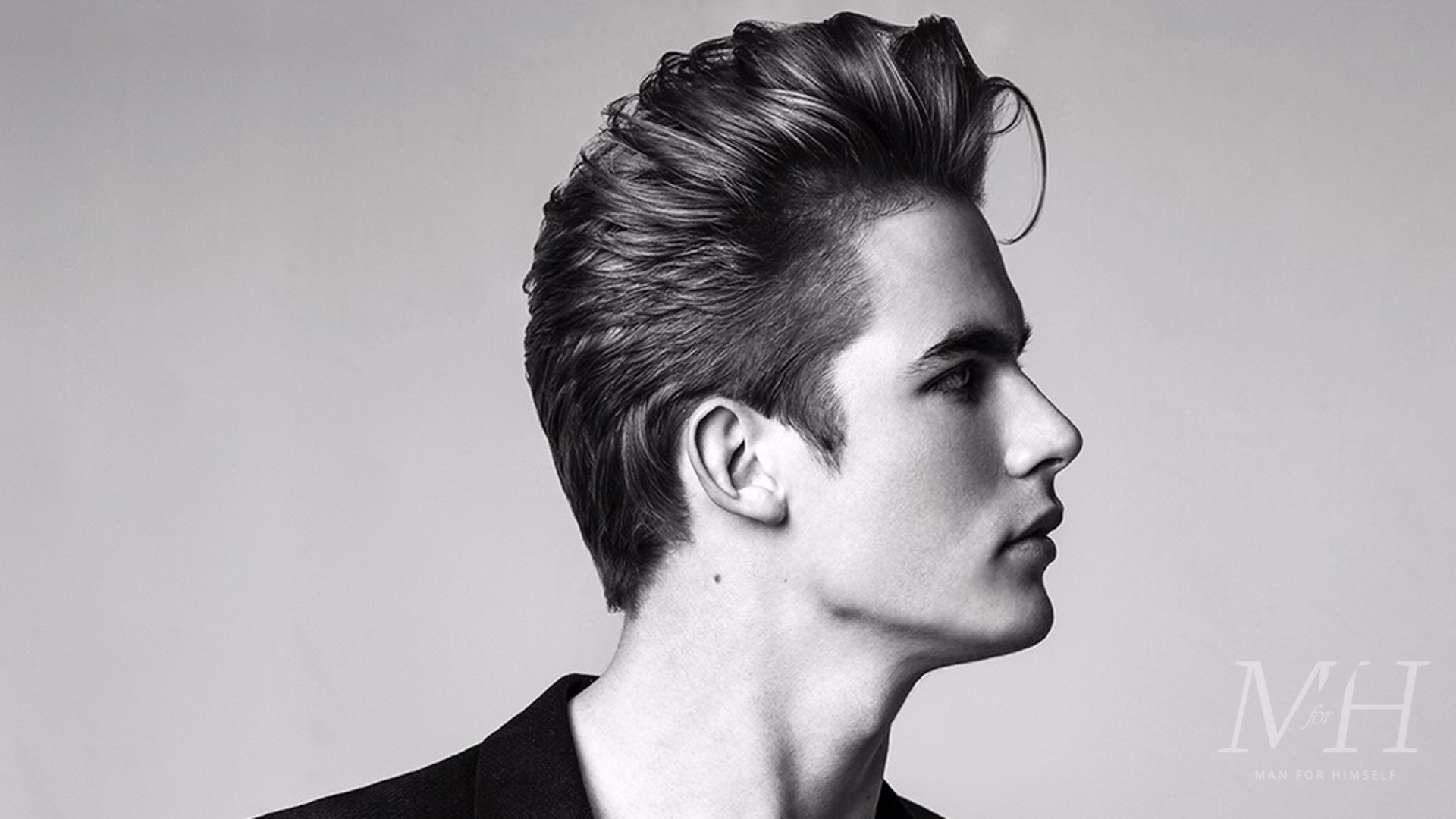This black-and-white profile photograph captures a young white male, likely in his late teens or early 20s. Only his head and the upper neck area are visible, with the image cutting off just at the start of his shoulders. His head is turned to the left, gazing away from the camera. His hair, a mix of brown with lighter tones, is voluminously styled in an Elvis Presley-like, old-school fashion, reminiscent of classic movie stars, complete with a spit curl. He has a straight, smallish nose and a mole behind his right ear. At the bottom right corner of the photo, the initials "MH" are visible. The entire image is rendered in shades of gray, white, and black.